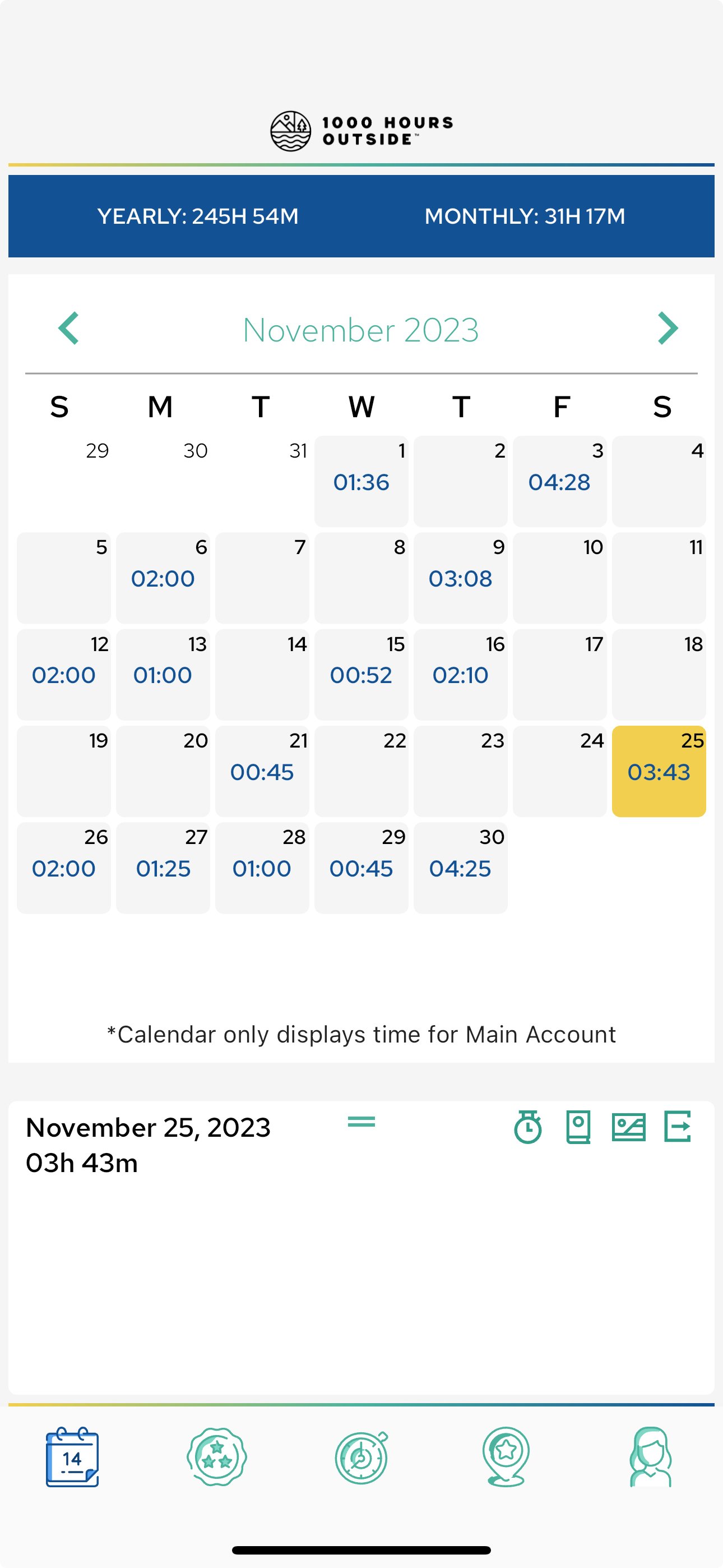The image depicts a detailed tracking calendar designed to monitor outdoor hours. At the top of the calendar, there is a circular symbol featuring a mountain above a body of water indicating the theme of outdoor engagement. Adjacent to the symbol is the text "1,000 Hours Outside," signifying the annual goal of spending a thousand hours outdoors.

Directly below this emblem, a blue bar displays cumulative tracking stats: 245 hours and 54 minutes of outdoor activity logged yearly, and 31 hours and 17 minutes for the current month. Beneath this bar lies the primary calendar interface, specifically set to the month of November, with navigation tabs available for switching between other months.

Each day within the calendar is annotated with the specific hours and minutes spent outdoors. Days without outdoor activity are left blank. An informational note below the calendar clarifies that the displayed time pertains only to the main account.

Additionally, a summary for November provides a detailed breakdown of daily outdoor hours. At the bottom of the image, there is a navigational menu, with the calendar currently selected. Other menu options are also visible, and the "Account" section is accessible on the far right side of this menu.